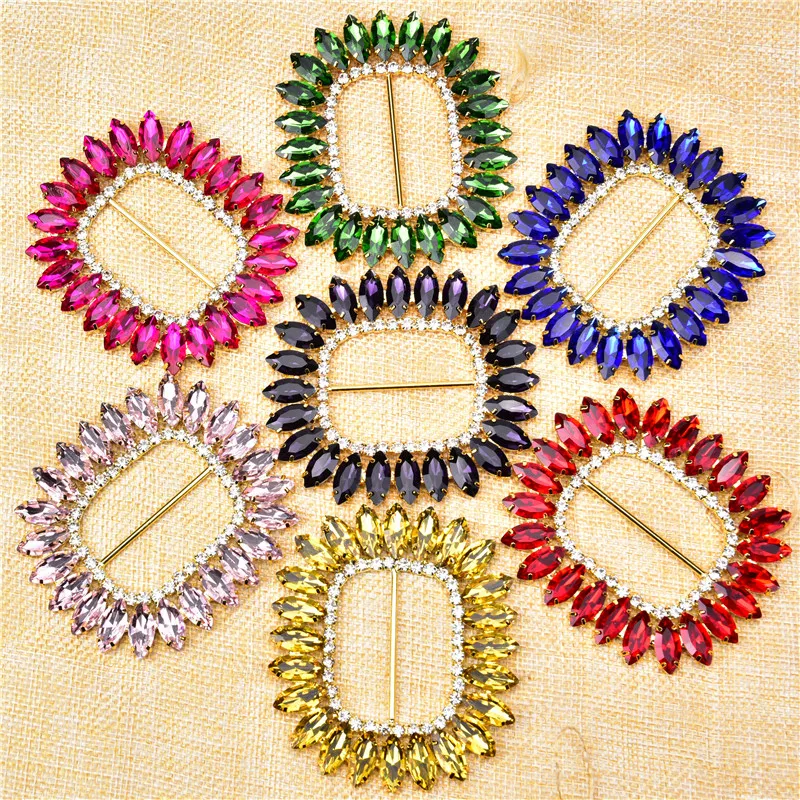In this detailed image, we see seven exquisitely arranged brooches, each featuring a distinctive array of vibrant gemstones. These brooches are placed on a beige, custard-colored fabric, forming a floral or clock-like pattern. The brooches are rounded square in shape and encrusted with small, colored gemstones around their perimeters, with dazzling diamonds on the inner sides of these gemstones. Each brooch has a hollow center, through which a golden pin runs horizontally.

Starting from the top (12 o'clock position) and moving clockwise, the brooches exhibit the following colors: a lush green (emerald) at the top, a deep blue (sapphire) to the upper right, a rich red (ruby) further down, a golden yellow (possibly citrine) at the bottom, a light pink stone, a darker pink (which might be a ruby or another pink gemstone), and finally a central brooch with a darker purple (amethyst) gemstone. Each gemstone appears to be calibrated and set to mimic jewels such as emeralds, sapphires, rubies, and amethysts, surrounded by sparkling crystal accents along the inner edges, lending an opulent, jeweled look to the brooches. The entire composition suggests both elegance and luxury, showcased perfectly against the soft, textured background.